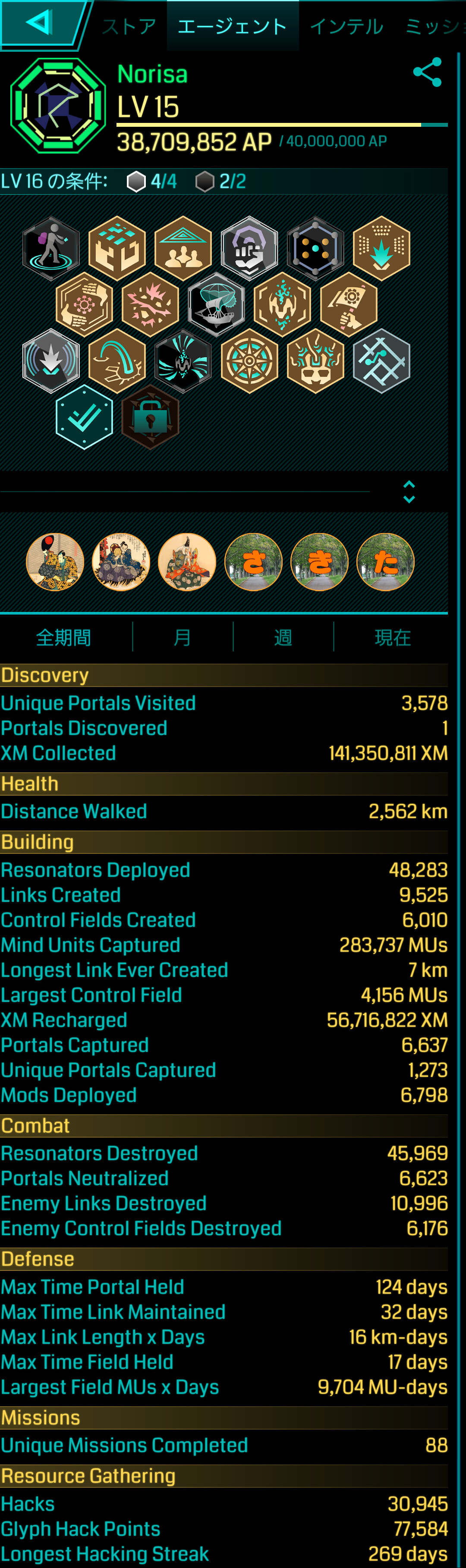This image is a detailed screenshot from a mobile device or a tablet, depicting a game interface with a black background. At the top, it prominently features the name "Narissa" in green, followed by "Level 15" in yellow, and the number "38,709,852 AP" which likely represents the player's accumulated points. The interface includes various icons and hexagon shapes that symbolize in-game items or achievements. The middle section displays numerous circle icons, possibly representing different game badges. Below these icons, there are yellow headers categorizing various player statistics, such as discovery stats, health stats, building stats, combat stats, defense stats, missions, and resource gathering. Under each category, blue text details specific game metrics such as unique portals visited, distance walked, resonators deployed, links created, control fields created, XM collected, the largest control field, and the longest link ever created. The screenshot encompasses the entirety of the image and includes text in multiple colors including black, light blue, brown, yellow, gray, orange, and red, possibly with some text in Japanese at the very top.